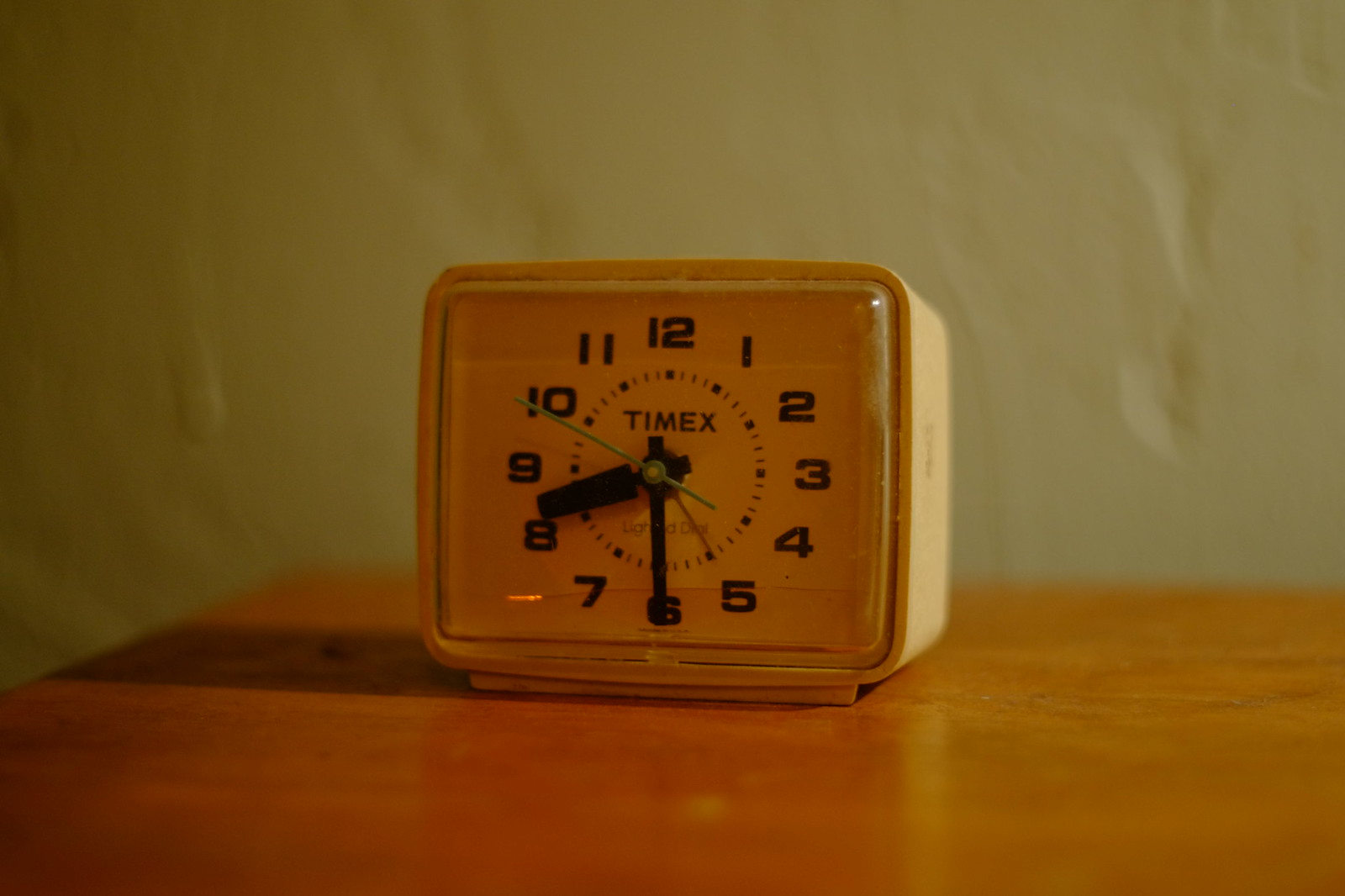In the image, there's a small, vintage Timex travel alarm clock set on the corner of a light-colored wooden bedside table. The clock, identified as the Cube 10 Timex model, displays the time as 8:30. Its body is a plastic, yellow or tan frame, and it has a white clock face with clearly marked black numbers and dots indicating the minutes around the perimeter. The hour and minute hands are black, while the thin second hand is green, which glows in the dark. The background features a textured wall appearing green in some descriptions and white in another, but generally noted to be unsmooth with divots, resembling wood.